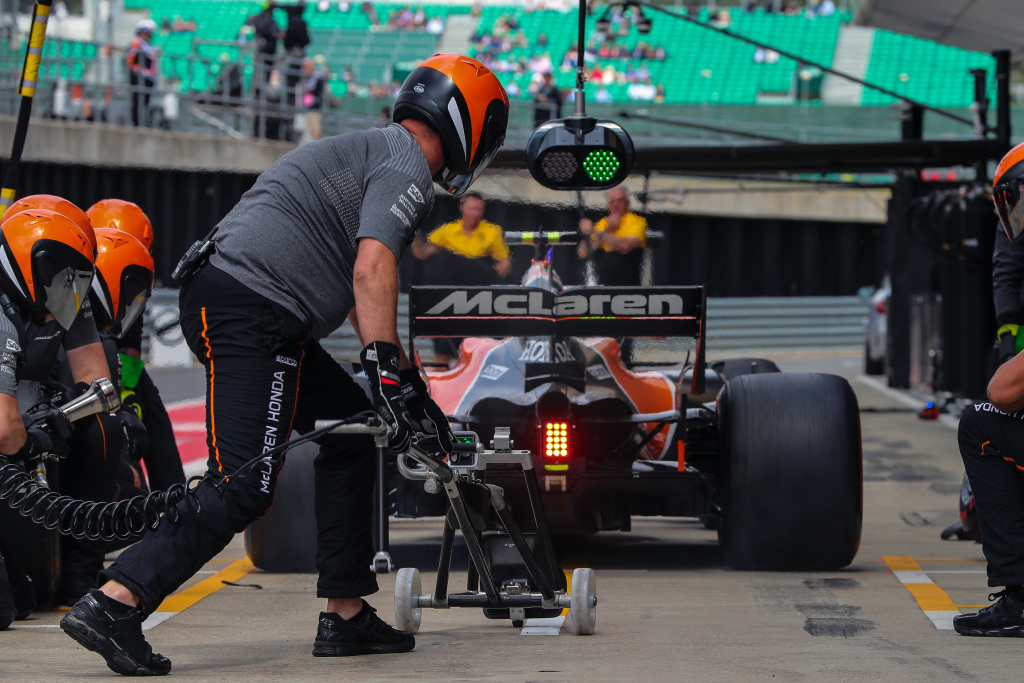In this daytime image taken at a racetrack, the scene is dominated by a sleek, orange and black McLaren race car situated in the pit stop area. Above the car is a stadium with sparsely filled green seats, and a closer viewing area with rails where more spectators stand. At the very top, a stoplight is flashing green, signaling "go." The race car's wing prominently displays the "McLaren" logo. Several crew members, identifiable by their orange helmets, are busy around the car. They appear to be performing diagnostics, changing tires, and other maintenance tasks. Notably, one crew member at the back of the car, dressed in black pants, a gray t-shirt, and black shoes, is holding a roller-like tool. The car itself features wide, low tires and a low-slung design indicative of high-speed performance.